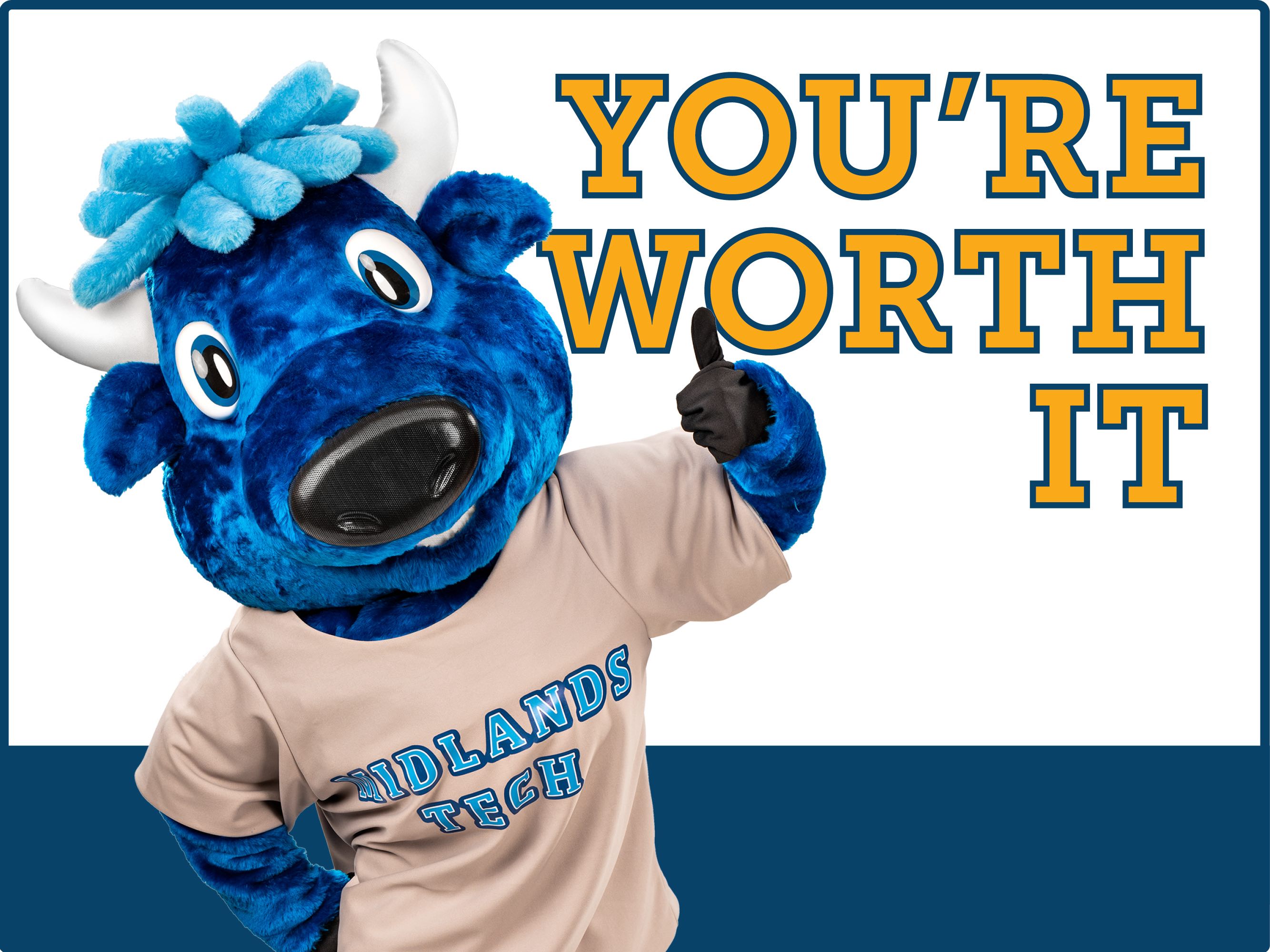This is a detailed poster for Midlands Tech featuring their blue bull mascot prominently on the left side. The mascot has a blue face, light blue hair, white horns, and big blue eyes with white centers. He sports a beige t-shirt that reads "Midlands Tech" in cyan letters with a white outline and a dark blue shadow. His expression showcases a bright smile with visible white teeth. The bull is giving a confident thumbs-up with his right hand, which is clad in a black glove, while his left hand presses against his shirt. In the top right corner are the words "YOU'RE WORTH IT" in bold, yellow font with a blue outline. The background of the poster is mainly white, with a dark blue stripe at the base, juxtaposed to the mascot’s vibrant blue tones.